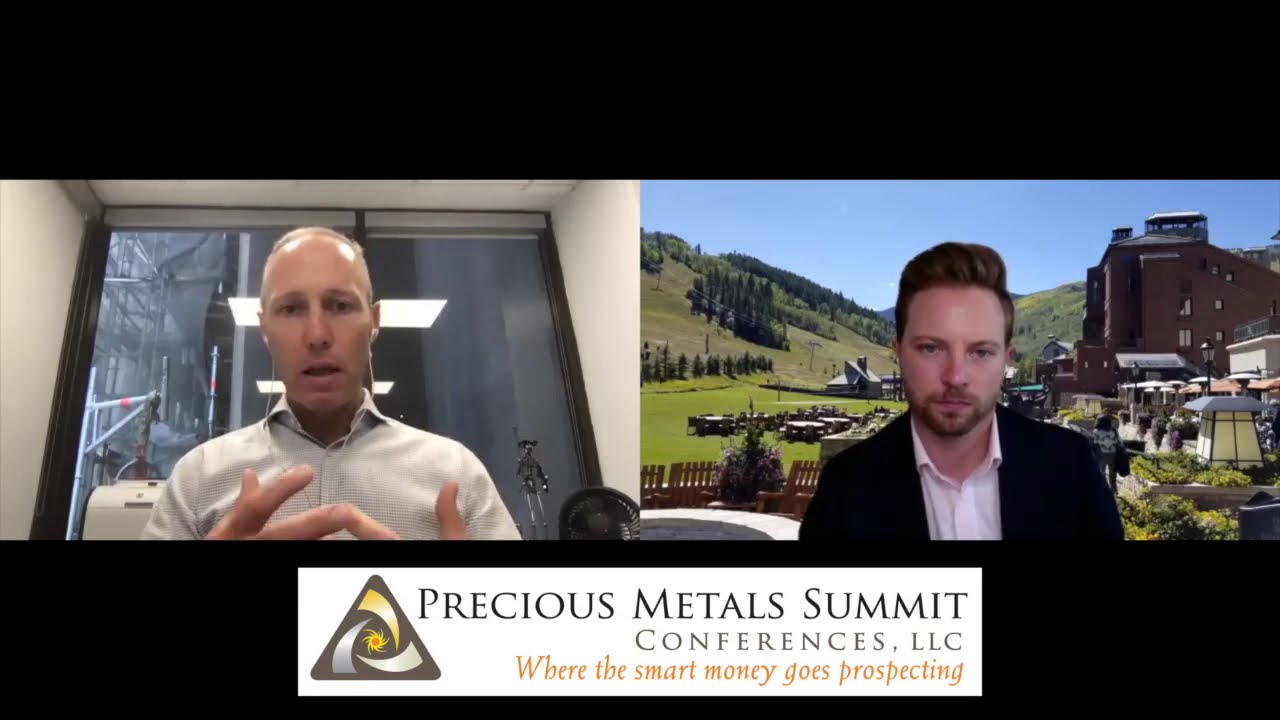The image is a detailed screenshot of a Zoom conference call featuring two white men. On the left, a man in his 40s to 50s with a buzzcut hairstyle and a white button-down shirt is speaking. He appears to be in a domestic setting, standing in front of sliding glass doors. On the right, another man with swooped brown hair, a beard, and a mustache is dressed in a black suit coat over a white shirt. He is using a virtual background depicting a summer mountain resort with hills, trees, and buildings. The screen is framed with black bands at the top and bottom, with the lower band featuring a white text box. This text box, along with a small triangle logo on the far left, reads “Precious Metals Summit Conferences LLC, where the smart money goes prospecting.” The overall impression is of a formal online conference or live stream.